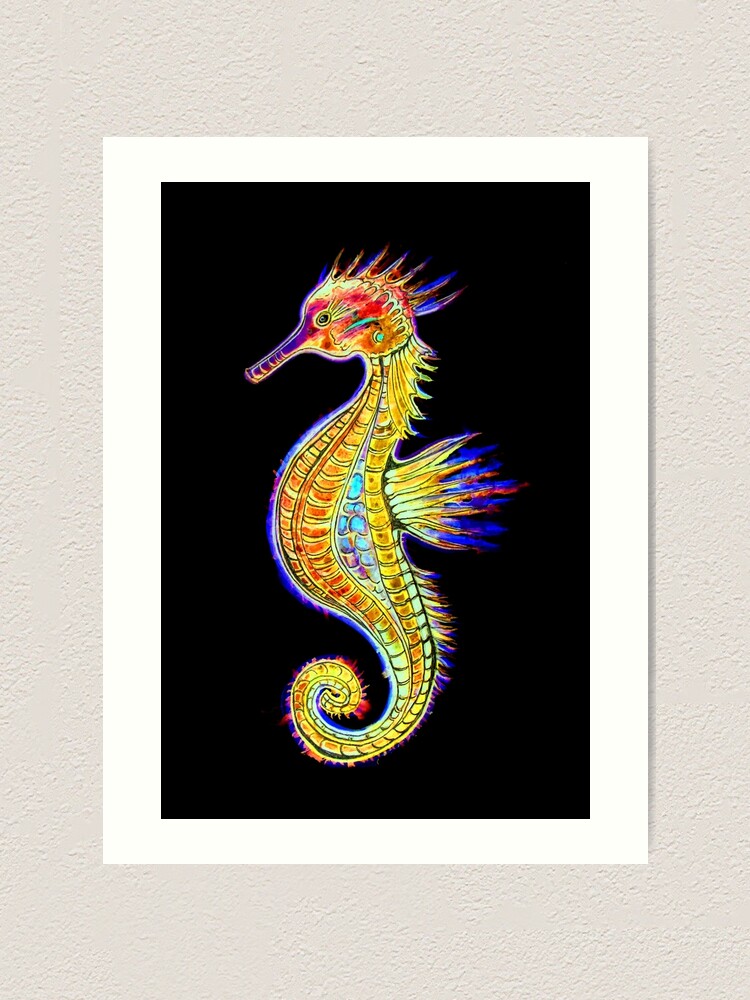This image features a vibrant art piece of a seahorse, showcased within a white paper frame against a black background. The seahorse, facing left, is an explosion of colors, including vivid blue, red, yellow, and turquoise. Its wings or fins seem to glow with a bluish hue, creating a striking outline. The head and chest of the seahorse are predominantly reddish, with turquoise scales adorning its midsection. Spikes can be seen on the top of its head. The entire piece appears to be rendered in a watercolor style, adding to its vivid and lively appearance. Additionally, the image includes a beige stucco wall behind the framed artwork, enhancing its display setting.